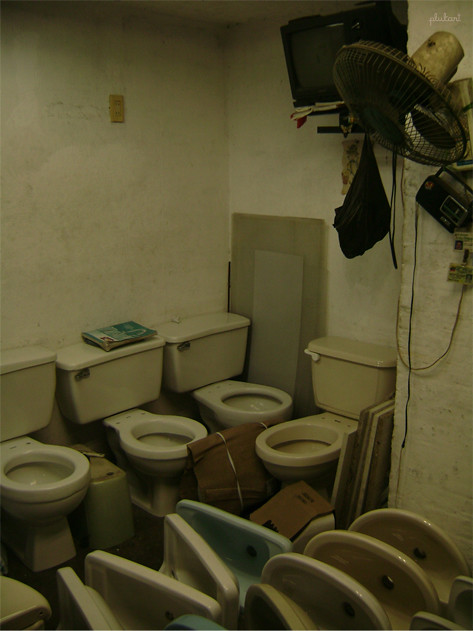The image depicts a dark, dingy room with dirty white brick walls, possibly an old repurposed classroom. In the upper left-hand corner, a thick television reminiscent of those from Channel One days is mounted on a stand. Below the television, the brick wall shows signs of wear, with either peeling paint or a hole. To the right, there is a large industrial fan with a crusty old handle, pointing downward from its perch on the wall. The room's lower section has several toilets: three lined up along the right-hand wall and one more on the back wall. The toilets appear unused and are without water, with lids unattached and set aside. Additional porcelain objects, possibly sinks, are scattered at the bottom left-hand corner, displaying a mix of rectangular and rounded bowls. Small plumbing fixtures and window screens can also be spotted among the restroom supplies. The overall ambiance is bleak and somewhat neglected.